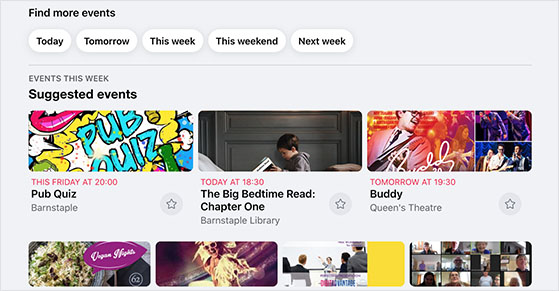A gray and light gray interface features predominantly black text, with highlighted sections as specified. Centered on the gray background, several white boxes provide event listings categorized by time frames: "Today," "Tomorrow," "This Week," "This Weekend," and "Next Week." The header "Events This Week" is rendered in bold gray font.

Highlighted in thicker, bolder text is a section titled "Suggested Events." The first event listed is a "Pub Quiz by Barnstable," set for this Friday at 8:00 PM. Directly below, an event labeled "The Big Bedtime Read, Chapter One" from Barnstable Library is scheduled for today at 6:30 PM, illustrated by an image of a child lifting the top of his desk in a classroom setting.

An aqua-colored note under the pub quiz listing features doodles and the words "Pub Quiz." The final visible event is scheduled for tomorrow at 7:30 PM: a discussion about Buddy Holly at Queens Theater. The remainder of the event list is cut off and not visible.